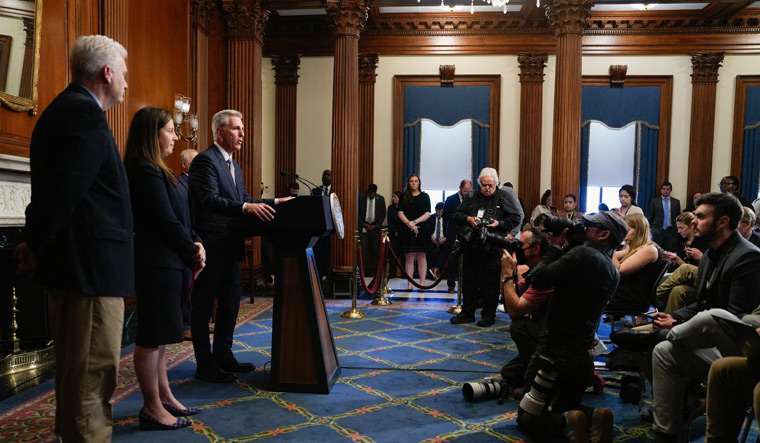This color photograph captures a press conference featuring former Speaker Kevin McCarthy, who stands at a podium flanked by a woman and two men, all dressed in formal attire. The event takes place in a stately, well-appointed room adorned with mahogany columns and wooden paneling. The elegant space also features blue and gold curtains with wooden trim on the windows, and is anchored by a decorative fireplace made of marble and brass. The blue carpet beneath them is intricately woven with green, red, and gold patterns. Surrounding McCarthy, photographers with cameras and journalists with notebooks are either kneeling or standing, capturing the moment. Behind them, an audience of seated men and women, along with additional men standing along the walls, are visible. The room’s refined atmosphere is punctuated by a red velvet rope at the back, enhancing the formal setting of this political event.